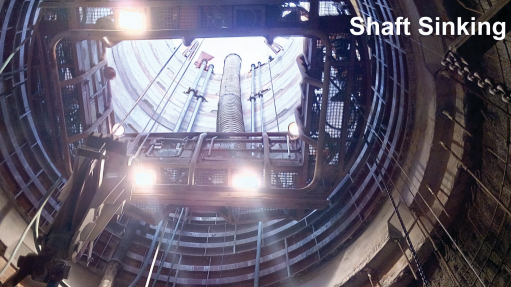The image depicts a view from the bottom of a cylindrical, circular structure that appears to be a construction site, possibly related to a reactor, shuttle, or dam. The scene features a mix of concrete and various metals, lending it a highly mechanical appearance. The structure, surrounded by metal tubes and numerous hanging cables, extends upwards towards an open top, where a bright white light from the sky is visible. Interior lights are pointed downward from the fixture, illuminating the area, and there appears to be some machinery, possibly an elevator platform equipped with chains and pulleys, which suggests that people can ascend and work within this construction. In the upper right corner of the image, white text overlays the scene with the words "shaft sinking," providing some context for the construction work being depicted.